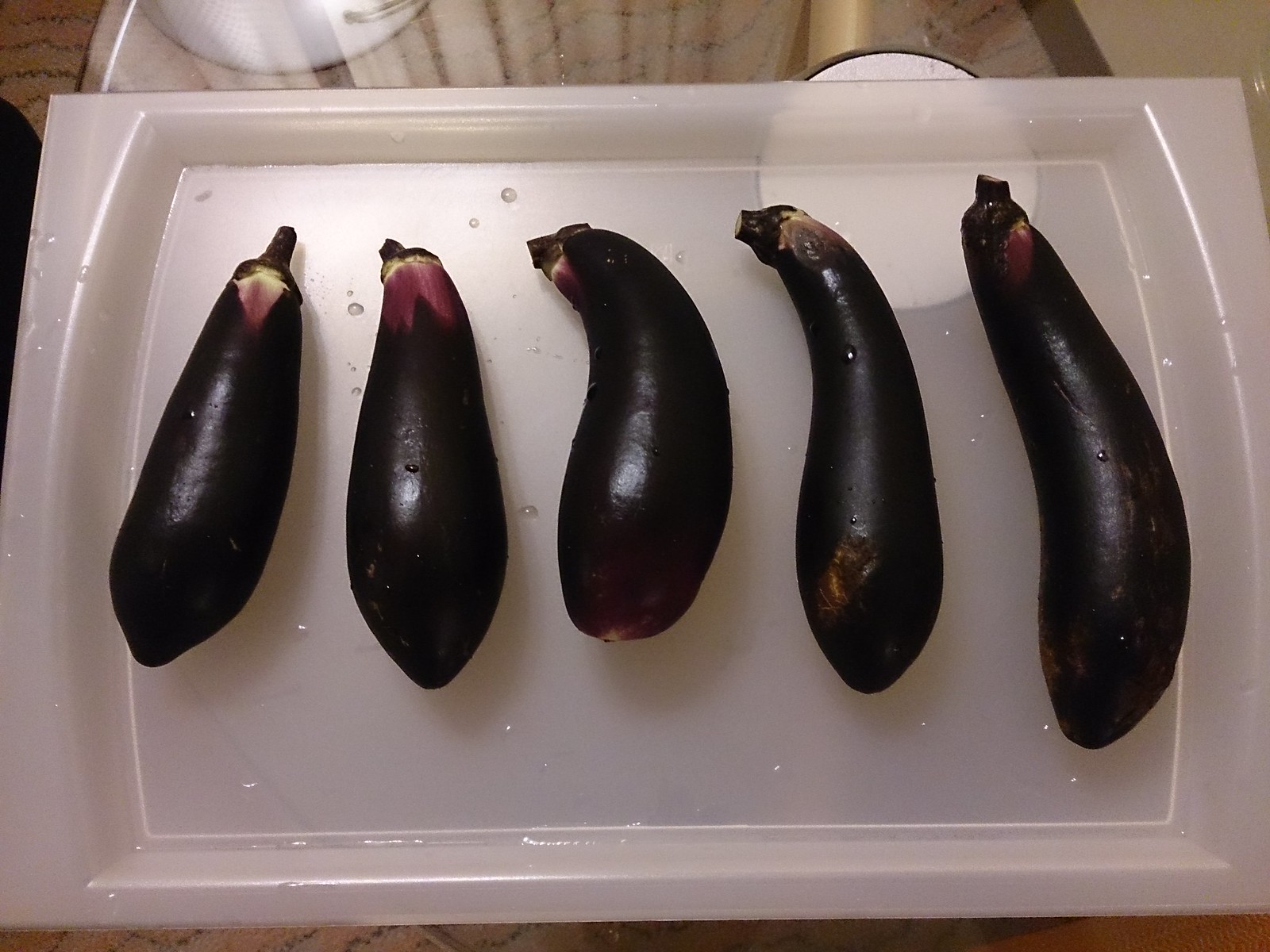This close-up photograph captures five freshly washed, deeply dark purple to almost black eggplants arranged side by side on a semi-transparent, rectangular white tray with beveled edges. Water droplets glisten on both the eggplants and the tray, indicating they were recently rinsed. The eggplants vary in length and curvature; the ones on the right are notably longer and more curved, while those on the left are straighter and slightly shorter, with the second and third eggplants being wider. The tray rests on a glass table, reflecting round, white ceiling light fixtures. In the top right corner, part of a wooden table texture is visible, adding an interesting contrast to the composition.